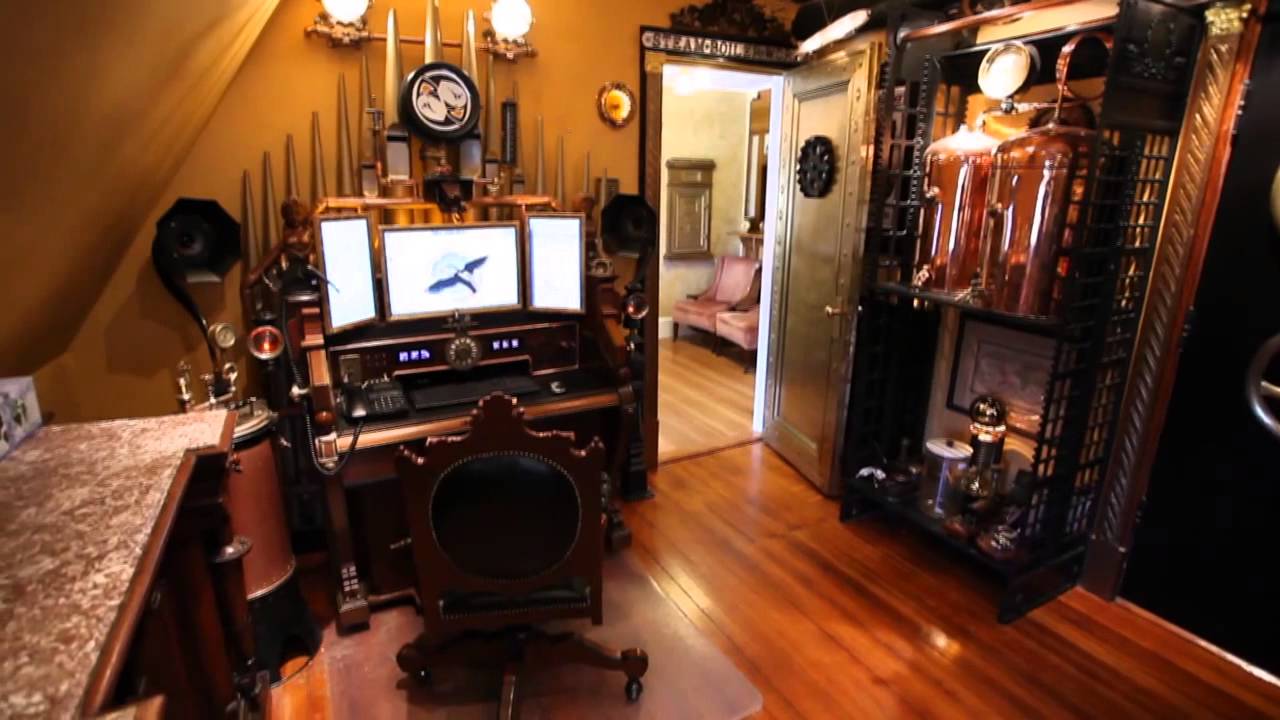The photograph captures a cozy office area within a residential environment, featuring a highly polished wooden floor that exudes warmth. The camera is pointed at a corner where on the left wall, an open doorway leads to another room, revealing more of the wooden flooring and two chairs in the background. Adjacent to this door is a unique workstation desk that resembles a pipe organ, equipped with three flat-screen monitors – one horizontal in the center and two vertical on either side. An ergonomically intriguing office chair sits in front of the desk. The right wall is adorned with a large shelf holding two prominent copper-colored, metal cylinders that appear to be alcohol distilleries, complete with gauges and possibly a brewing station setup. The shelf also contains a variety of other shiny, glass-like objects. In the far left corner, an old-style sound horn extends from a cylindrical device, adding to the room's vintage charm. The walls exhibit a warm brownish hue, and the ceiling is fitted with lighting, completing the inviting indoor ambiance.